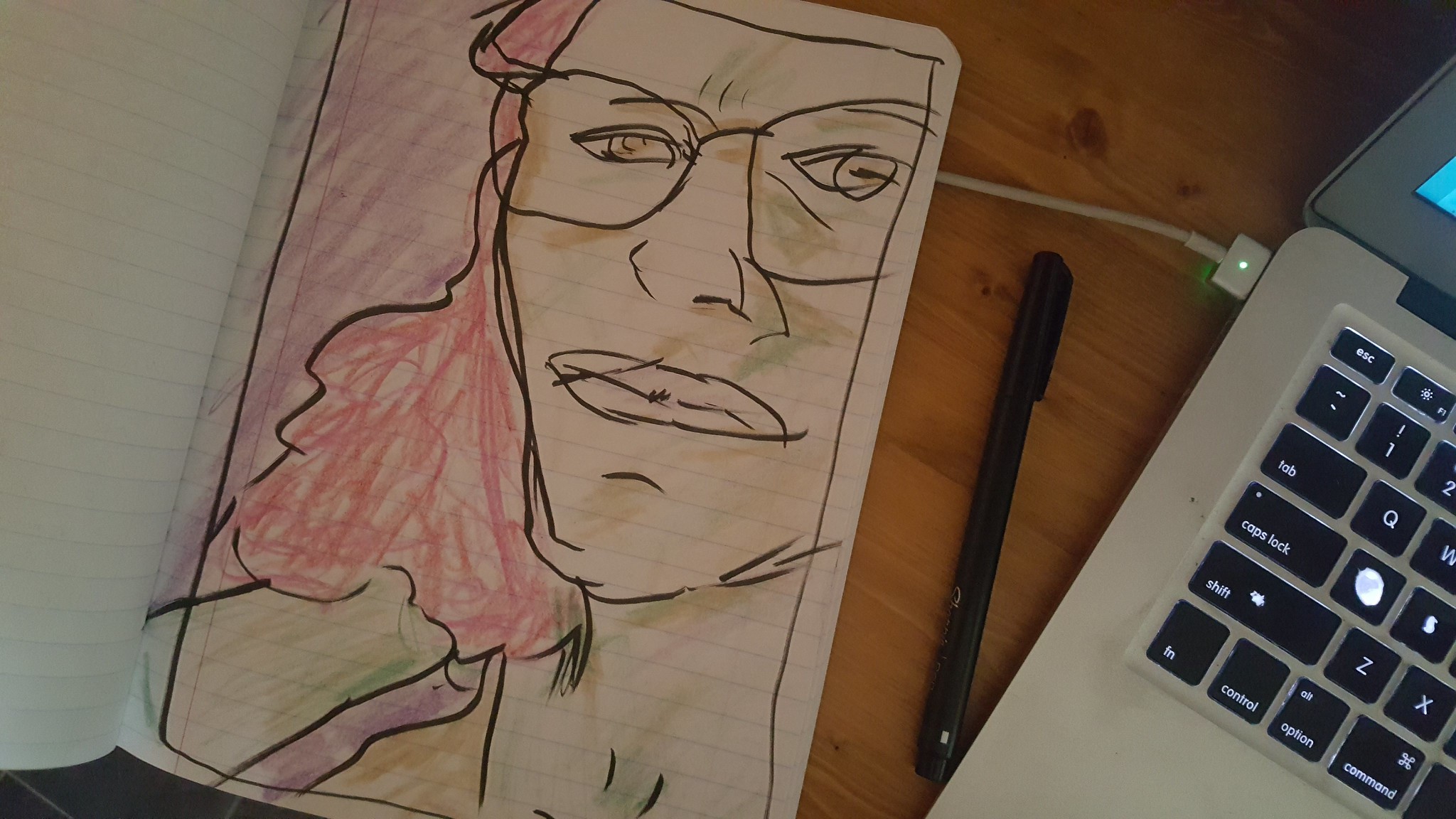The image depicts a scene on a brown hardwood table. On the left side, there is an open notebook, with the left page blank and the right page featuring a detailed pen ink drawing bordered in black. The drawing is a headshot of a person with a pronounced chin and larger nose, who is wearing black glasses and has long, vibrant pink (alternatively described as red hair drawn in marker). The person's clothing, in hues of purple, green, and yellow, stands out against a background with purple and green colors and, according to one description, purple bottom trim on a wooden floor. Next to the notebook, positioned centrally, lies a black pen. To the right of the pen, a silver MacBook is seen with the charging cord plugged into the upper left-hand corner. The MacBook has a gray bezel, black keys, and the visible corner of the screen displays a turquoise color.